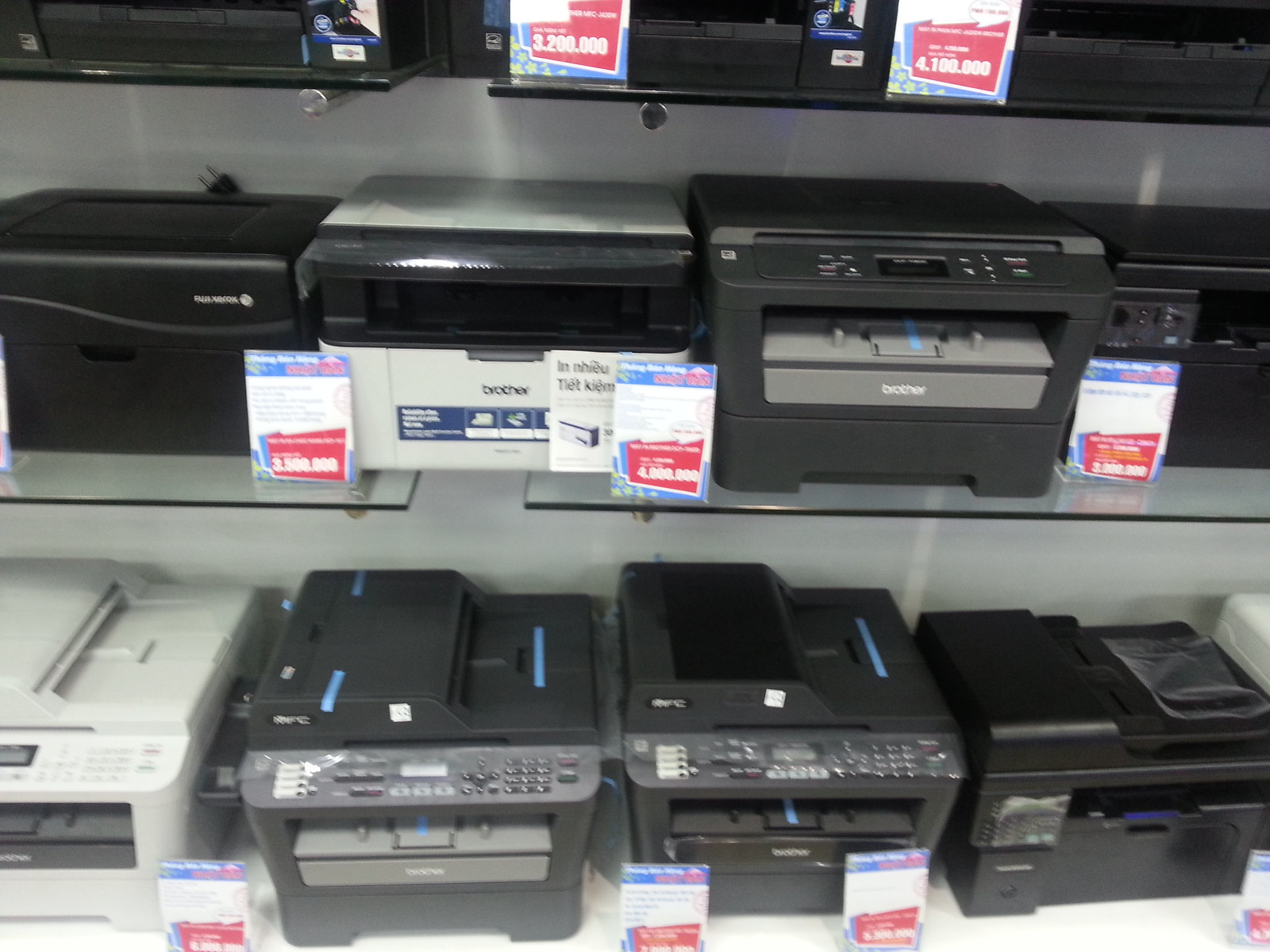This image shows a display in an electronics store featuring multiple shelves stocked with various printers. There are three visible shelves, although the top shelf is partially cut off. Each shelf holds a mix of printers, primarily featuring Brother brand models as indicated by the visible logos. The printers are mostly black or black and gray, with a few exceptions in whitish gray and two-tone colors.

The top shelf, partially visible, seems to contain mainly black printers. The price tags on these items are hard to decipher due to the blurry quality of the image and the possibility of being in a different language, but numbers like "3.200.000" are discernible.

On the middle shelf, there is a noticeable mix of black and gray printers, with price tags indicating a range between approximately 3.5 to 4 million in the unclear currency. 

The bottom shelf displays the largest printers, which appear capable of additional functions like photocopying and scanning. These also include mostly black models with at least one white printer on the left, and seem to be priced higher, around 6 to 7 million, albeit the exact currency remains indistinguishable. Overall, the entire setup suggests a variety of all-in-one printers are on offer with various price points emphasized in bold but blurry text.